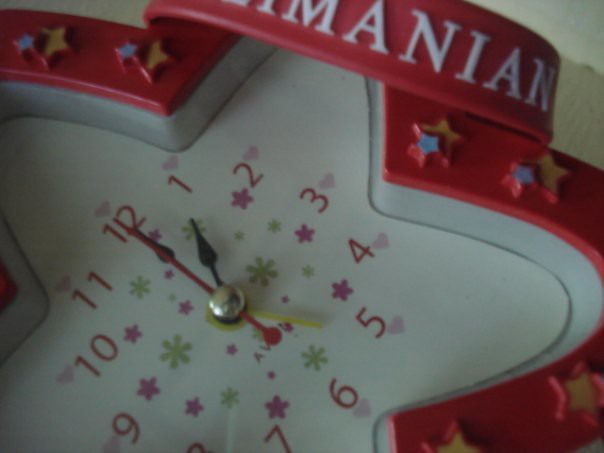The image shows a close-up view of the central portion of a children's star-shaped clock. The clock's outer frame is red, embellished with small yellow and blue stars. The main face of the clock is white and decorated with green and pink flowers, as well as heart shapes that represent the numbers 1 through 12. The clock features black hour and minute hands, a red second hand, and an additional yellow hand with an unclear function. At the center, there is a silver ball pivot point. The time displayed on the clock is 1 o'clock. Surrounding the clock's edge is a band with partially visible text, showing the letters "MANIAN," though the full word remains unknown.